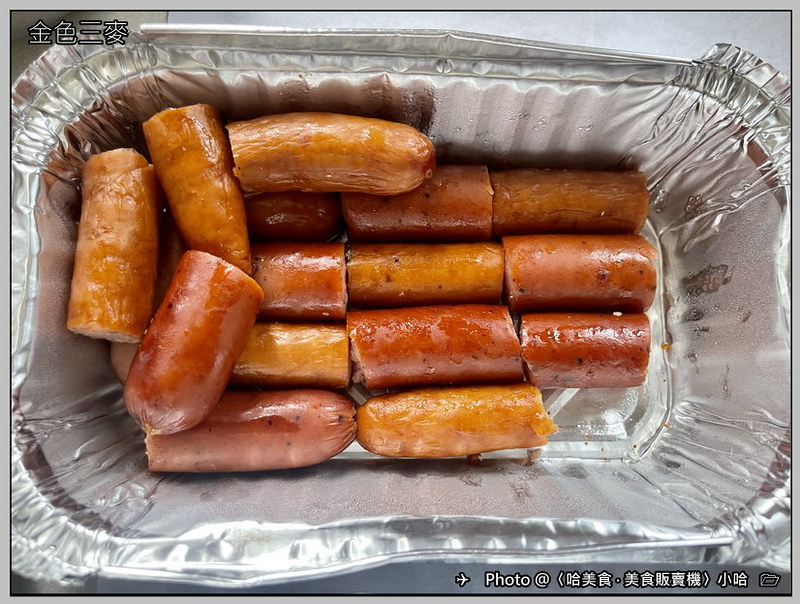The image depicts an aluminum disposable pan with sides that come up, containing several sections of cooked sausage links. The sausages, reddish-brown with a shiny, smooth surface and slightly shriveled from cooking, have a hot dog-like texture and resemble breakfast or summer sausages. The presence of condensation along the rims of the pan suggests that the sausages were recently cooked, possibly barbecued or oven-baked. The metal pan is placed on a gray tiled surface, evident from the visible grout lines. Notably, the image includes Asian writing in the upper left and lower right corners, with the latter accompanied by the word 'photo' and a silhouette of an airplane, suggesting a photo credit in what appears to be Japanese script.